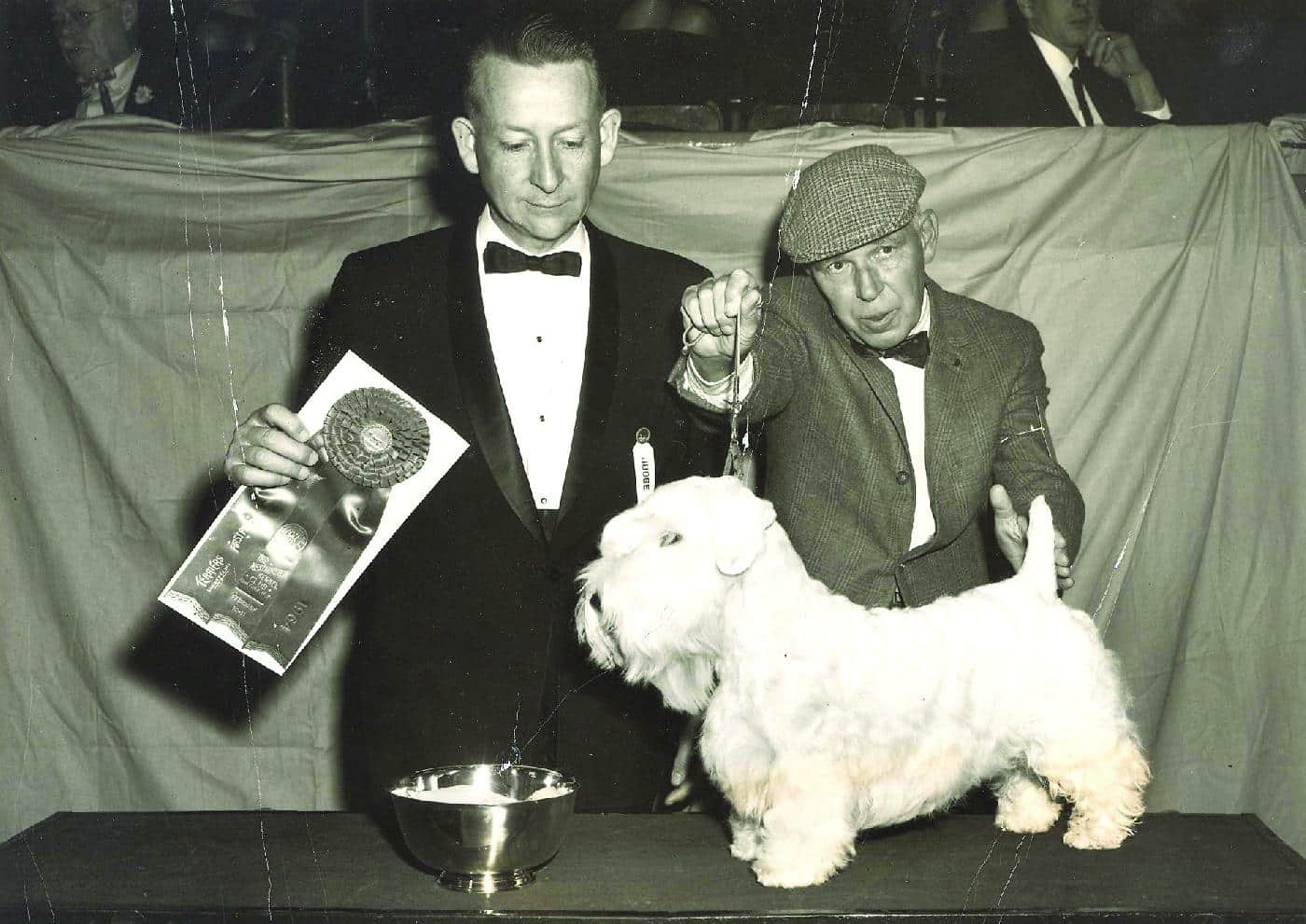This black and white photograph, slightly worn with age, captures an elegant moment from a dog show decades ago. At center stage, a small, white, fluffy dog, reminiscent of a schnauzer or terrier, stands on a table with a rectangular head, beard-like facial hair, short stubby tail, and a small bowl of white substance in front of it. Two men stand behind the table: the one on the left, possibly a judge, is dressed in a refined tuxedo with a black bowtie, holding a ribbon and gazing down at the dog. The man on the right, presumably the handler, is shorter and attired in a plaid suit, bow tie, white shirt, and a pageboy cap, holding the dog's leash. Both men form a scene that suggests the dog has just won an award. In the background, partially obscured by what appear to be curtains or sheets, there is a glimpse of an audience wearing suits and ties, watching the proceedings attentively.